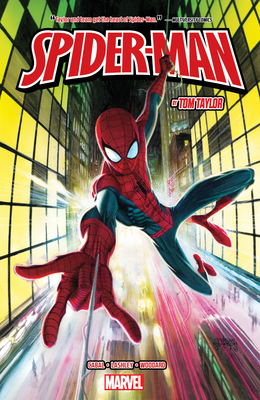The image is a digital screenshot of a vibrant comic book cover featuring Spider-Man prominently in the center. Spider-Man, adorned in his classic red and blue suit, swings dynamically towards the viewer, his hand outstretched with thumb, index, and pinky fingers extended as he shoots his webs. His mask has white eye lenses outlined in black. The background showcases a cityscape with tall buildings on either side, their windows glowing in yellow and green hues. Below, motion-blurred traffic including a bus and several cars indicates the bustling city beneath him. At the top, a red and white logo reads "Spider-Man" with "Tom Taylor" listed as the author. Smaller, less legible text and the Marvel logo appear at the bottom. The cover is filled with a diverse palette of reds, blues, yellows, greens, and accents of pink, black, and gray.